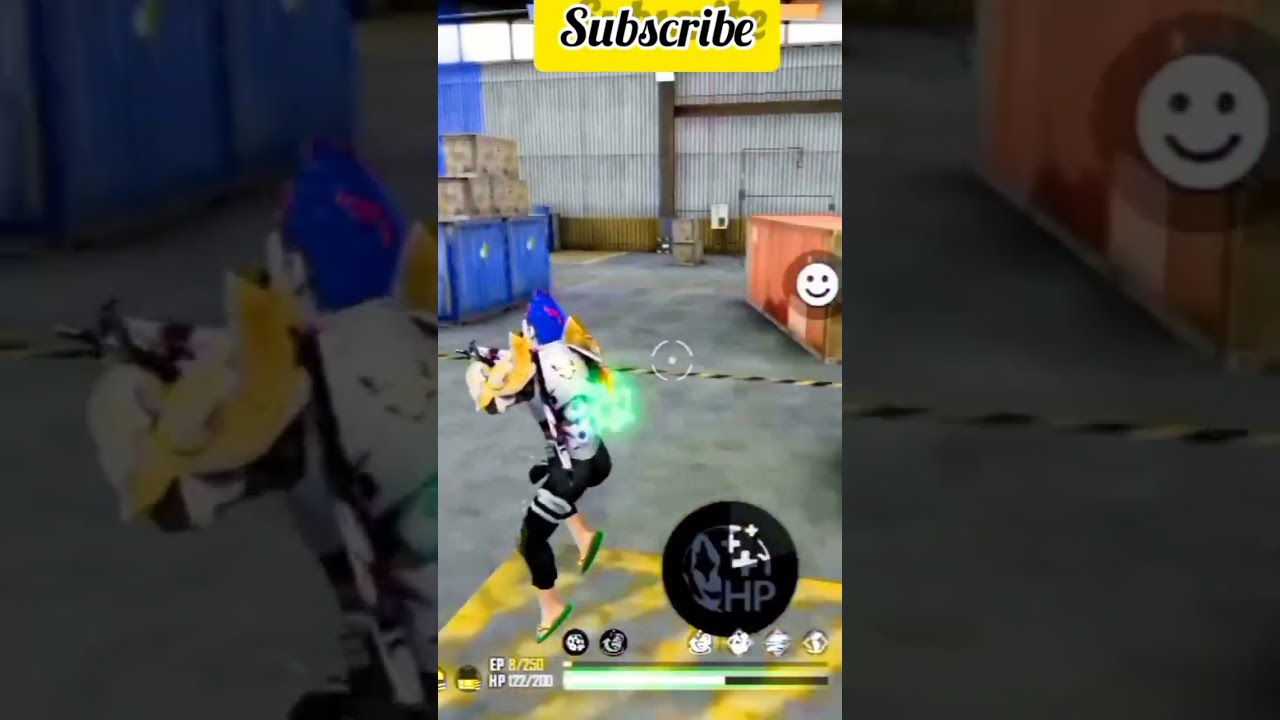This image is a detailed screenshot of a mobile video game, likely set inside a warehouse with metal framing and upper windows. Dominating the scene is a 3D character with blue hair, wearing body armor that includes yellow shoulder pads, black pants, and green flip-flops. The character appears to be holding or pointing an automatic rifle. The warehouse setting also contains blue storage bins and brown boxes stacked on crates, visible against a gray pavement floor.

At the very top of the image, a yellow rectangle with black text outlined in white prominently displays the word "subscribe." This call to action is positioned centrally. At the bottom of the image, there are gameplay indicators, including an HP meter reading "HP 122-200" and possibly an EP meter for experience points. 

Additionally, a white smiley face with black eyes and a black smile is seen on the right side of the image, set against a translucent gray or black background. Yellow paint marks the floor, emphasizing the warehouse or possibly parking lot theme further. The overall image composition suggests this is part of a video game competition or a gameplay channel that viewers are encouraged to subscribe to.